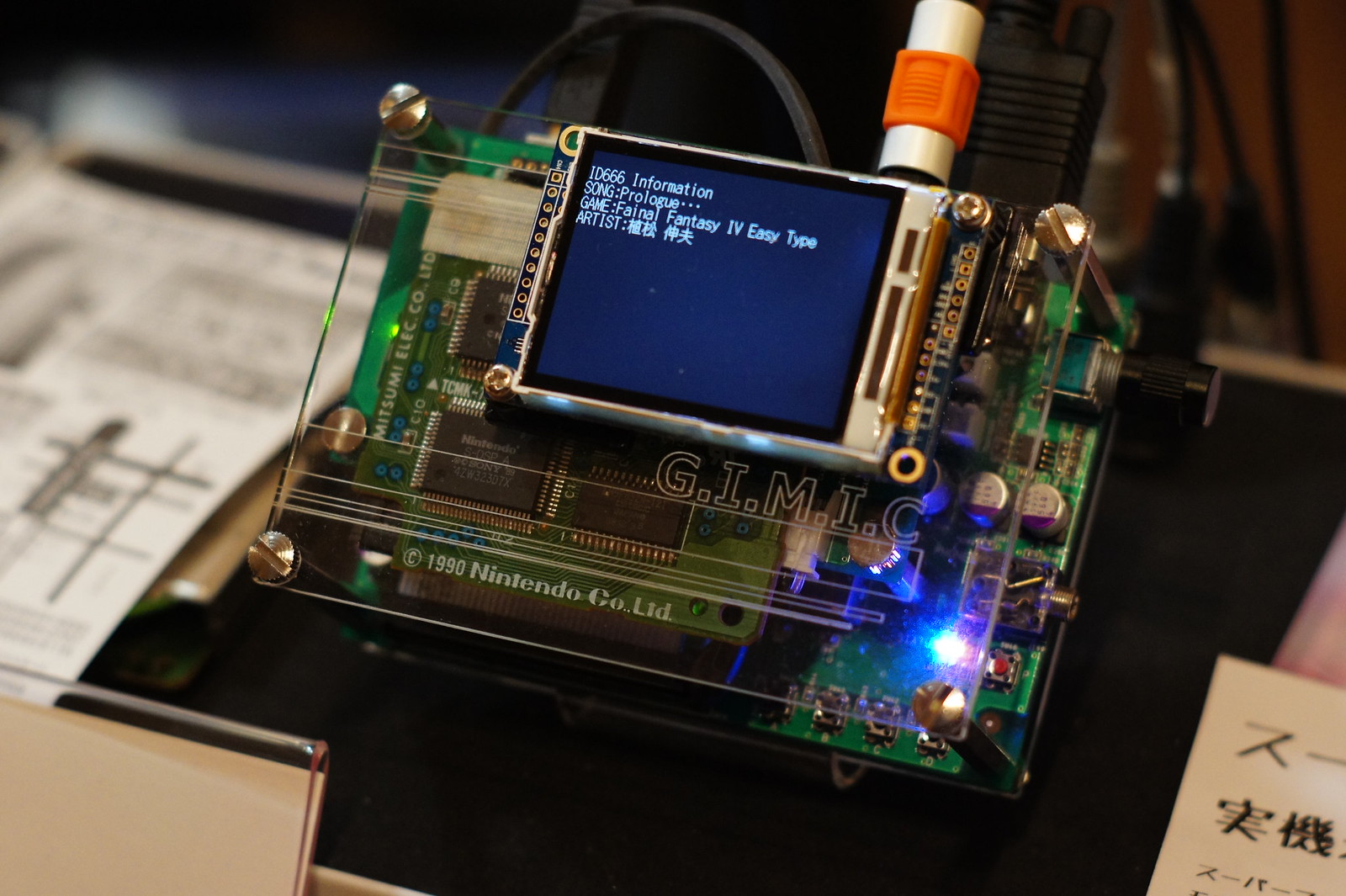The image features a zoomed-in view of an electronic device, resembling a computer circuit board or motherboard, encased in a clear plastic or glass cover. The cover prominently displays "GIMIC" in all caps, possibly denoting an acronym, and "copyright 1990 Nintendo Co. Ltd." A small LCD screen is mounted on the front of the device, displaying white text on a black background. The text reads: "ID 666, information, song, prologue, game, Final Fantasy IV, easy type, artist" followed by Japanese characters for the artist's name. The device appears to be some form of museum piece, as indicated by the visible corner of a sign or plaque in the bottom left. It is situated on what looks like a desk or table, with some papers nearby and cords visible in the background.